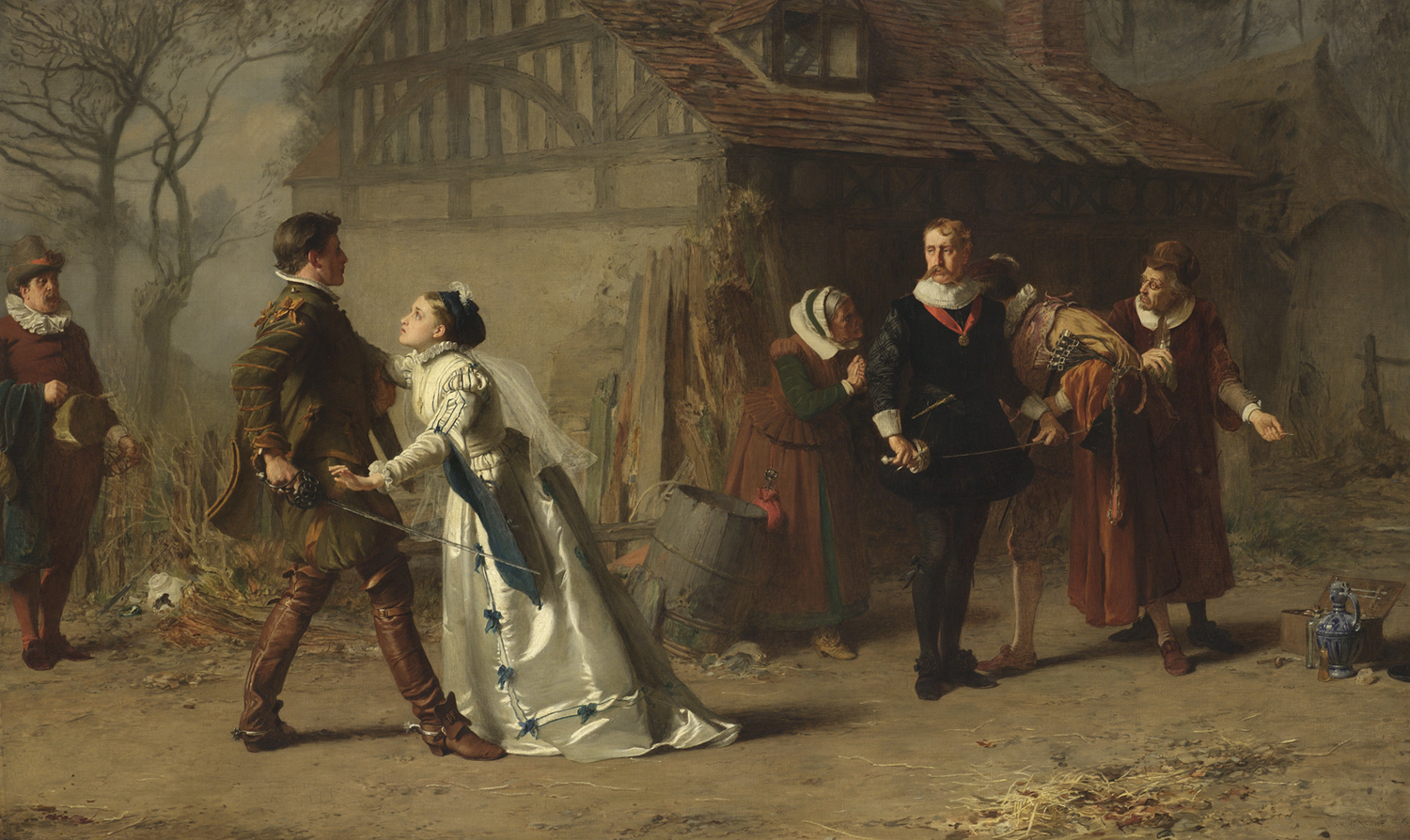The image is a classical painting set in what appears to be the 1800s, with a rustic, wooden barn and a barren tree in the foggy background. The scene is detailed with a dark, earthy brown palette, accentuated by deep burgundy and dark green hues. It depicts a dramatic confrontation: a younger man, adorned in a green jacket with gold fringe, brown leather boots, and a white collar, is held back by a woman in a pristine white gown. Her elegant attire includes features reminiscent of the period, such as bustles. She appears to be restraining him from engaging in a duel with an older man, dressed in somber black clothing and black shoes, complete with a white collar and a gold-handled sword. The older man has a mustache and is being conversed with by a small group of concerned onlookers—two men and a woman. Additionally, a man behind the younger man holds his hat, while another figure, obscured slightly by the fog, watches the scene unfold from a distance, adding depth to the painting. The composition, colors, and intricate details contribute to its antiquated and evocative atmosphere.